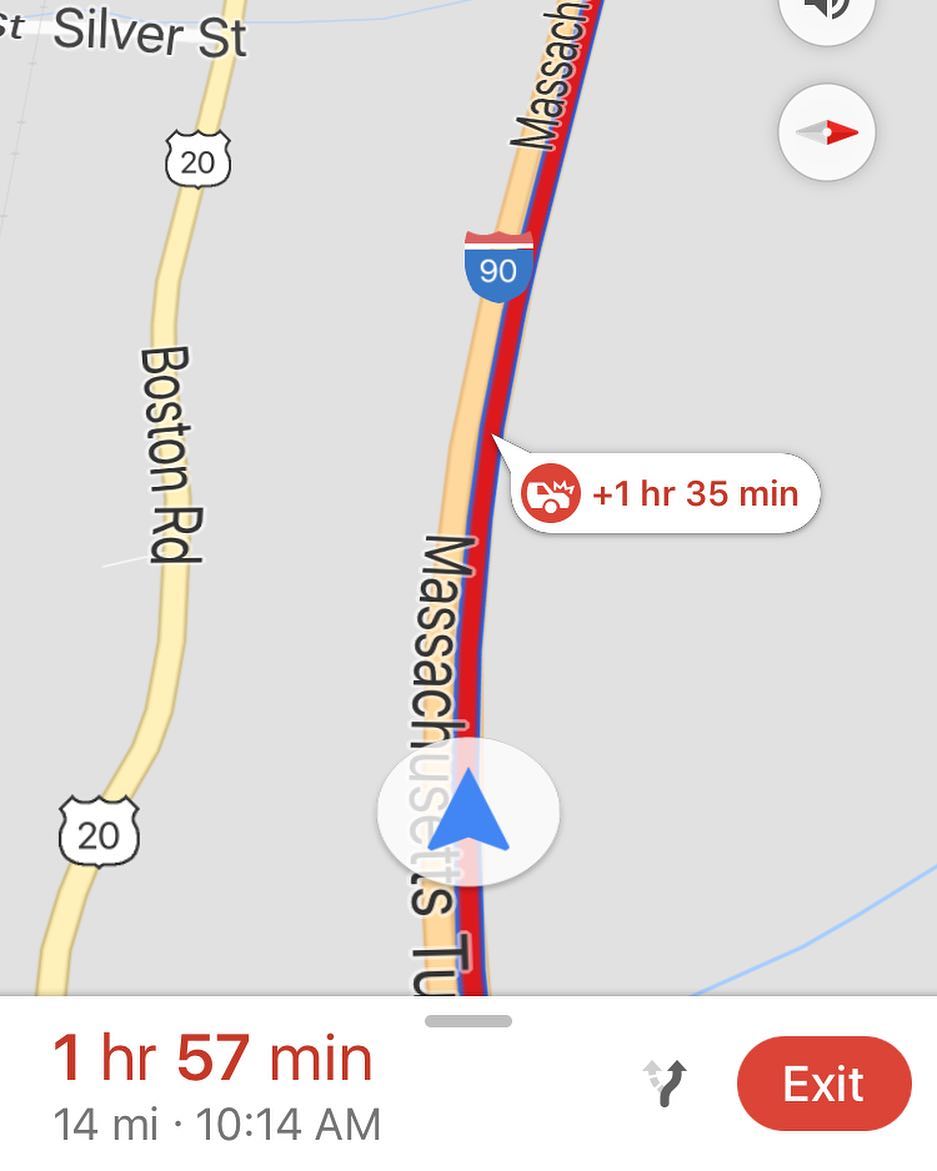### Caption

This image is a screenshot from a map application displaying a section of the Massachusetts Turnpike against a gray backdrop. The Turnpike, marked as a two-tone tan and red road, begins at the center of the image and extends upwards, curving slightly to the right. Directly parallel to the Turnpike runs Boston Road, a tan-colored route labeled with the number 20 in black text.

The Massachusetts Turnpike is clearly congested, as indicated by the red segments and a notification of a car accident causing an extensive delay of 1 hour and 35 minutes. The text "Massachusetts Turnpike" is prominently displayed in black font on the highway itself. The opposite lanes of the Turnpike are marked only in tan, indicating smoother traffic flow in that direction.

A compass symbol at the bottom of the image shows north pointing to the right. In the upper right-hand corner, a half-visible speaker icon implies voice navigation is active. Additionally, a message indicates an expected travel time of 1 hour and 57 minutes to cover a distance of 14 miles due to the traffic conditions. A red exit marker is situated at the lower right-hand corner of the image.